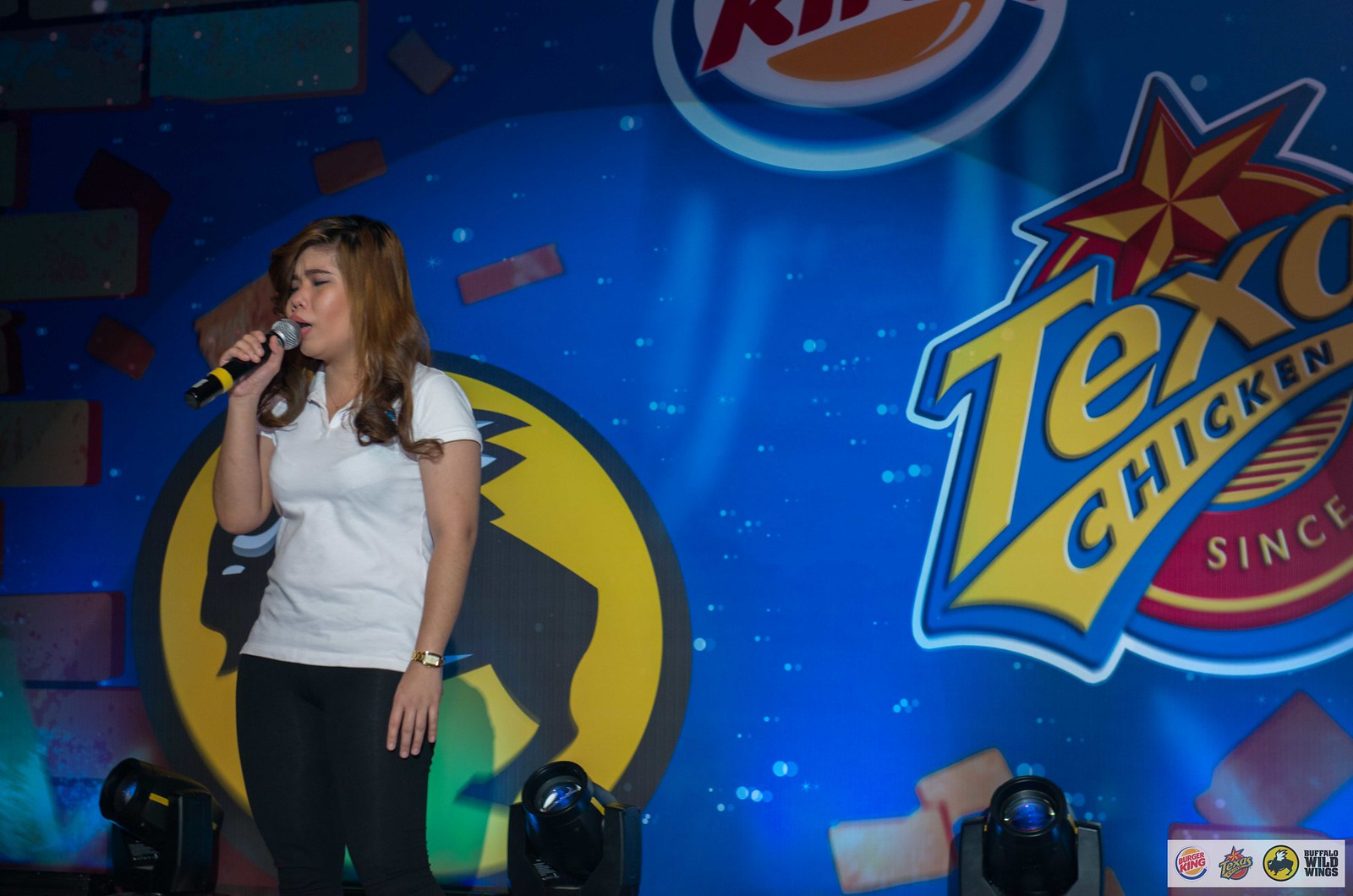In this vibrant image, a woman stands on stage, possibly singing or performing stand-up comedy, holding a black microphone with a red top close to her mouth. She is dressed in a white short-sleeved collared shirt paired with black pants and wears a watch on her left wrist. Her brown hair, reaching just past her shoulders, is illuminated by a spotlight. The backdrop behind her is a large blue banner adorned with multiple logos, suggesting a sponsorship by several brands. Prominently featured are a red and yellow star with "Texas Chicken" inscribed beneath, and the recognizable Buffalo Wild Wings logo, a black circle with a yellow interior. To the side, there's an additional logo with partial visibility showing letters like “K” or “R” and orange semicircles. The scene is accented by foreground spotlights pointing toward the audience, contributing to an engaging light show. Additional smaller logos for sponsors such as Burger King and Texas Chicken are also seen at the bottom, reinforcing the event's sponsored nature.